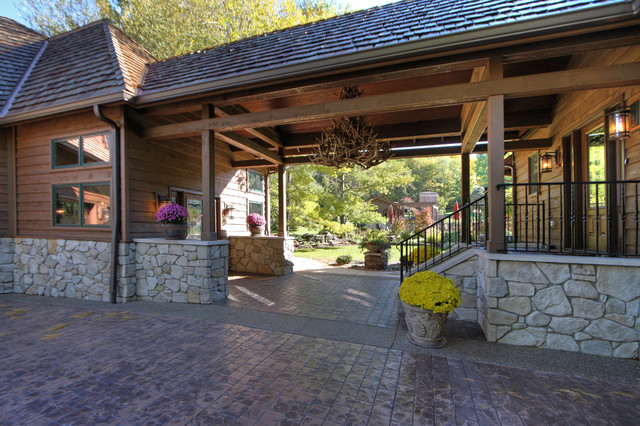In this image, we see a sunny, outdoor entrance to a nature retreat or a lodge. The structure features a combination of wood paneling and a gray stone facade that covers the lower portion of the building, complemented by a tan tiled roof. The entrance itself is marked by a brick road or driveway that has distinct brick patterns leading up to the building. Flanking the walkway are large stone flower pots with vibrant yellow flowers, and wooden pots containing fuchsia and pink flowers on either side of the entrance. A notable centerpiece within this entryway is a chandelier designed to resemble antlers.

The building includes glass windows set in a light tan frame with stone trimming around the edges. There's a black railing leading up a few steps to the right side of the entrance, while the left side is level with the ground. In the background, a wooded area with thick trees surrounds the property, and a grassy field is partially visible, dotted with red umbrellas covering outdoor tables. Additionally, there are lamps on either side of the doorway, adding to the rustic charm. The overall atmosphere is serene and inviting, with sunlight illuminating the distant landscape while the entrance remains shaded.